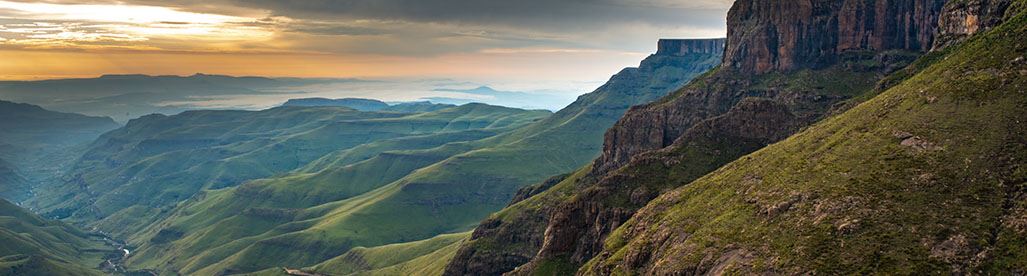The image is a panoramic color photograph of the Draco Mountain Range in Africa, captured in landscape orientation. The right-hand side of the image prominently features a rocky hillside with dark brownish-green cliffs and an olive-green layer of either moss or grass. These cliffs jut dramatically from the hillside. In contrast, the left side descends into a valley with gray-green grassy slopes that gradually decrease in elevation toward the horizon. Lower in the valley, there's a possible brook or creek, and along the horizon line, there might be a body of water or the illusion of clouds seen through different elevations. The photograph appears to be taken from atop a hillside, looking out across a range characterized by numerous peaks and valleys. The sky in the background showcases a stunning sunset with an array of colors: light yellow and orange near the horizon, transitioning to dark gray clouds higher up. The style of the image embodies photographic representational realism and captures the landscape during daytime.